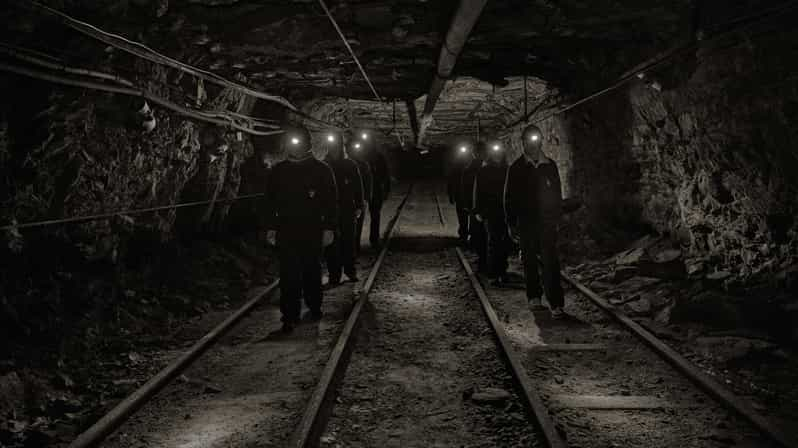In this striking black and white photograph of an underground tunnel, we observe a compelling scene of what appears to be a mine shaft. The image features two parallel railway tracks running through the tunnel, which are covered in dirt and flanked by walls encrusted with rocks and soil. Along these tracks, eight figures—presumably workers—are seen walking in formation towards the camera. Each worker on the left track and most on the right track wears a helmet equipped with a shining headlamp, casting a bright, white light that cuts through the darkness. Interestingly, the third man on the right track seems to be without a helmet and flashlight. The tunnel's walls and roof are adorned with an assortment of pipes and overhead wires, contributing to the industrial atmosphere. The horizontal orientation and the perspective view of the tracks narrowing into the distance enhance the depth and complexity of the scene, capturing the rugged essence of underground labor.